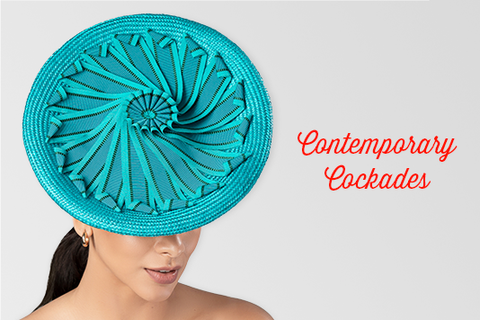The image features a woman with a long, dark ponytail, adorned with an eye-catching, oversized circular hat or cockade. The hat is a striking turquoise color, characterized by a large, round outer edge intricately woven with thin blue lines. In the center of the hat is a smaller raised circle, connected to the outer ring by twisted fabric strands that create a whirlpool effect. Adding further detail, the top of the hat showcases light blue, almost aqua ribbons with black stripes at the ends, forming a floral pattern. The woman's face is partially visible, showing only from the tip of her nose down to her pointy chin and shoulders. In red cursive letters, the words "Contemporary Cockades" appear on the right side of the image, set against a bright gray background, further emphasizing the striking design of the hat.